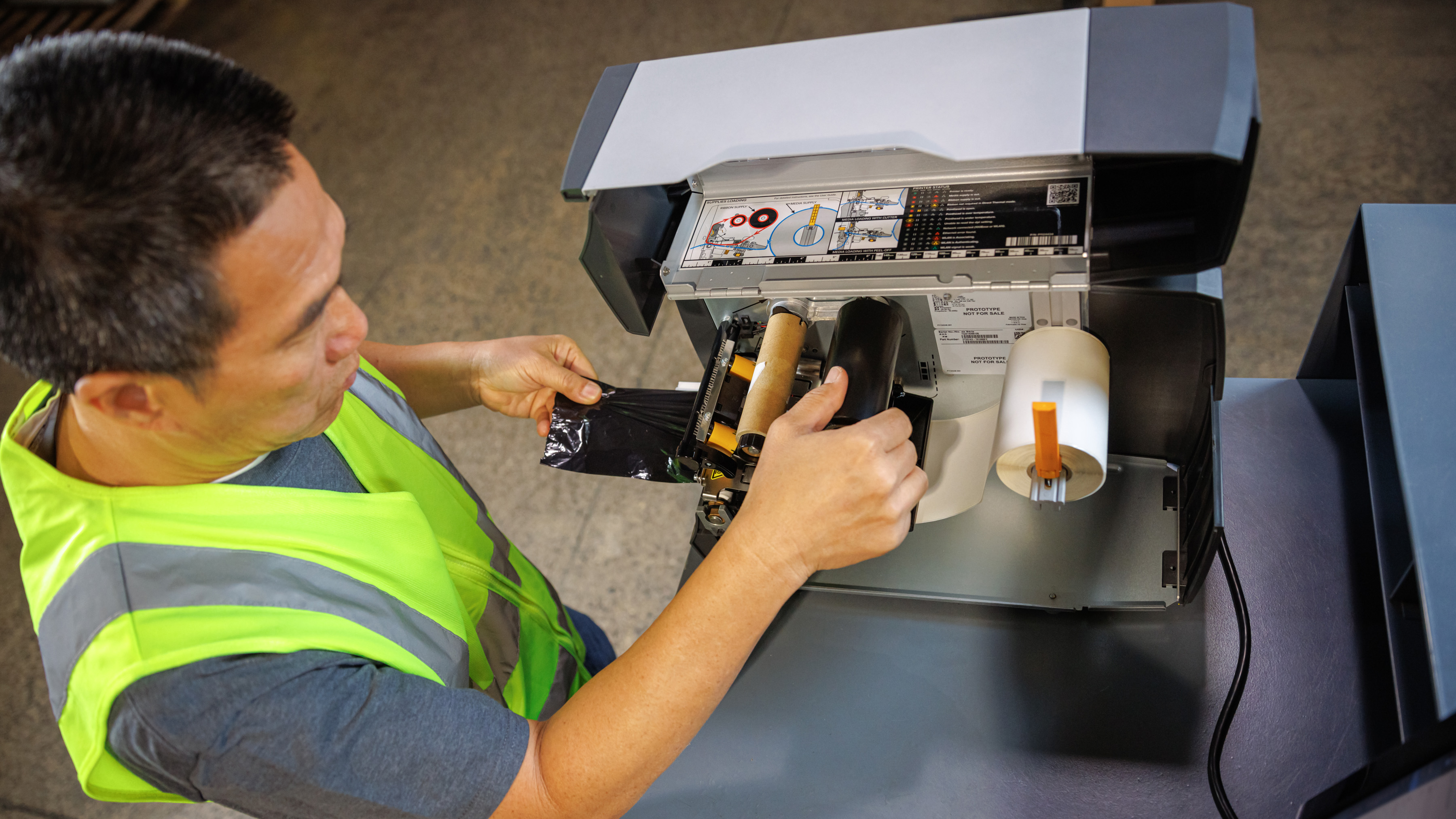The photograph is a color image taken from an overhead angle, capturing an adult Asian male wearing a reflective neon yellow vest with gray striping over a gray t-shirt. Positioned on the left-hand side of the image, he is engaged in operating a partly open machine. This device, potentially a prototype printer, has a mix of metal and plastic components, including a notable large electrical cord. The man is manipulating a black element with his left hand and a black cylinder with his right, seemingly ensuring the proper setup or refilling of the device. A white spool of paper and two rollers are visible, with a label near the white roller indicating "prototype not for sale." The machine’s gray, rectangular body has an exposed side, revealing internal mechanisms, while a yellow mustard-colored plastic component is positioned to the right, possibly holding the white spool in place. Despite the detailed view, the precise function of the device remains ambiguous, though it bears resemblance to a receipt printer. The man’s focused expression suggests he is either testing, demonstrating, or refilling the equipment while referring to an instructional label inside the case.